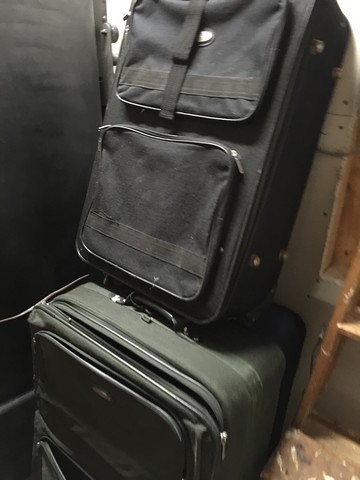This photo captures a tightly confined space with poor lighting, featuring a white shadowed wall in the background. To the right of the image, a wooden table leg or possibly a chair is visible, suggesting the presence of furniture. Central to the composition are two pieces of luggage: a large, thick, dark green suitcase positioned on the floor, and atop it, a slightly smaller black suitcase. The black suitcase, which features two sizable front zipping compartments, appears to be leaning back against the wall. To the left of the suitcases, there is a large black metal object, potentially a fridge or similar container. Although parts of the scene are partly obscured, the overall atmosphere hints at the interior of a storage or warehouse-like setting. No text or words are visible in the image.